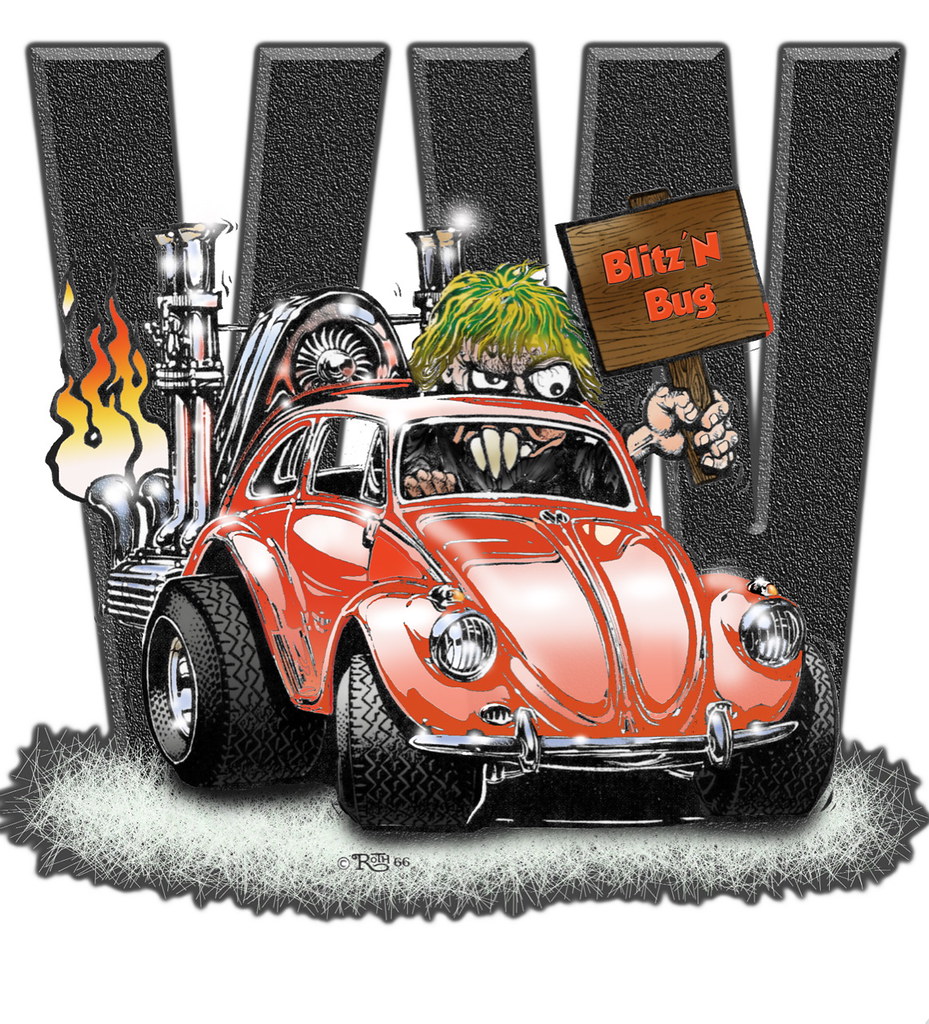This detailed illustration, a blend of hand-drawn art and digital manipulation, prominently features a souped-up, red Volkswagen Beetle. The Beetle, drawn with exaggerated, wide tires and a massive engine fitted at the back, expels visible flames and fumes. The background showcases large grey "VW" lettering, emphasizing the Volkswagen theme. Inside the Beetle sits a monstrous character with bulging eyes, green and yellow curly hair, and three downward-pointing large teeth. The character, holding a sign that reads "Blitzenbug," adds a whimsical, almost comic-book-style element to the scene. The image's collage-like composition, with shiny highlights and grey scribbled areas, enhances its vibrant and dynamic appearance, making it look like a sticker one might find in an auto shop.